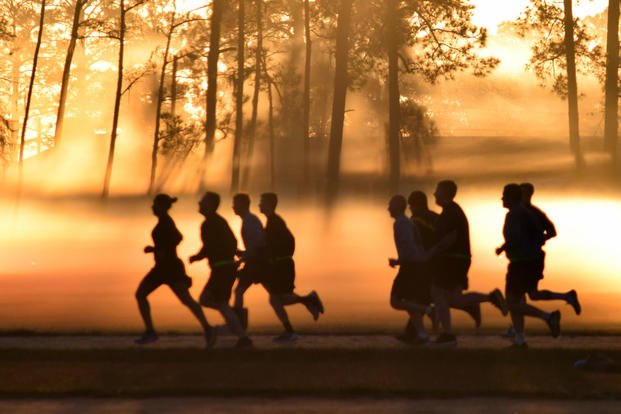This color photograph captures an early morning or late evening scene, bathed in the warm, hazy glow of an orange and pink sunrise or sunset. The focal point is a group of eight or nine runners silhouetted against the radiant sky, creating a striking contrast. The runners, mostly depicted as dark silhouettes, include a woman leading the pack with her hair tied in a bun, followed closely by several men. The group is split into two segments: a leading pack of four runners, with a noticeable space behind them before the following five. They run along a road or sidewalk flanked by grassy edges, set within a park or beside a forest. The backdrop features tall, thin trees, some bare and others with sparse foliage, adding to the serene yet dynamic atmosphere. The photograph's overall effect is a blurred motion of orange and brown hues due to the interplay of light, fog, or possibly smoke, contributing to the image's ethereal and motivational quality.